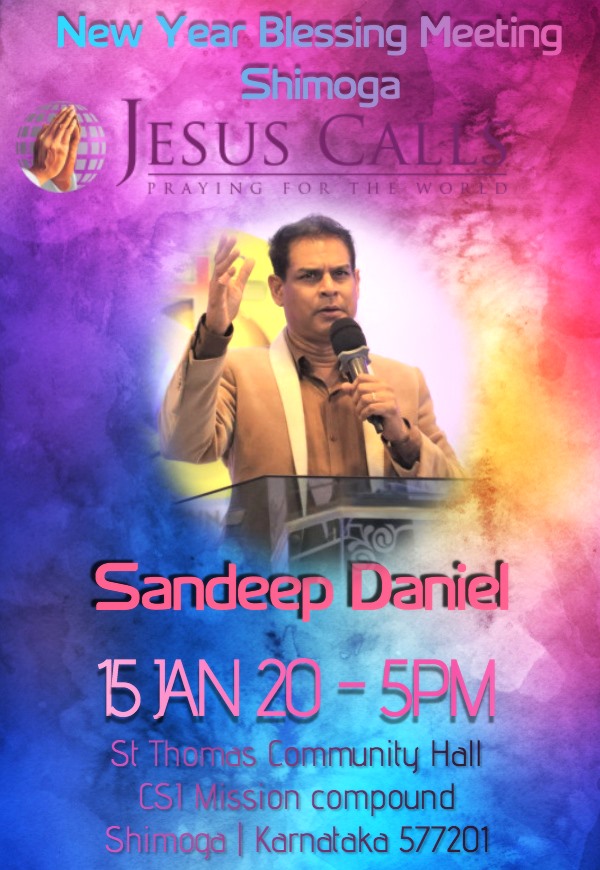This is a vertically aligned rectangular image serving as an advertisement for an upcoming religious event. The vibrant background features colorful clouds in hues of pink, purple, and blue, creating a visually striking backdrop. At the center of the image stands a man at a podium, engaged in preaching. He has short brown hair, a serious expression, and wears a brown suit jacket with a matching button-down shirt. His right arm is raised in the air, and he holds a microphone to his mouth with his left hand, emphasizing the action of speaking. 

At the top of the image, centered in bold blue letters, the text reads "New Year Blessing Meeting," followed by "Shimoga." Beneath, in large, capitalized purple letters, "JESUS CALLS" is prominently displayed and underlined, with the smaller phrase "Praying for the World" positioned just below. To the left of "JESUS CALLS" is a circular icon depicting two praying hands over a globe. 

Centered below the speaker, in large pink letters, is the name "Sandeep Daniel." Further down, it details the event date and time: "15 Jan 20-5 p.m." Lastly, the venue information is provided: "St. Thomas Community Hall, CSI Mission Compound, Shimoga / Karnataka 577201." All textual details are centrally aligned in the bottom portion of the image.